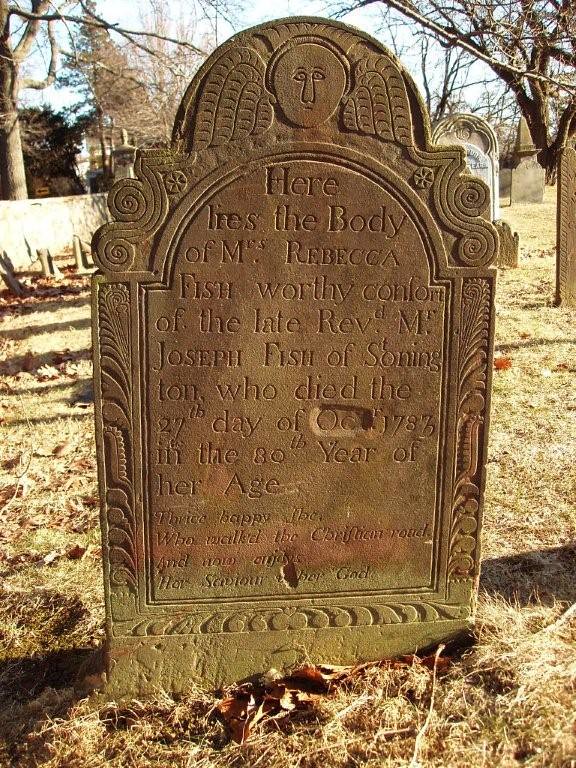The image is of an intricately designed headstone situated in an old graveyard, captured during a cool day either in the fall or winter. The scene is enriched with various trees, many bare or adorned with brown, falling leaves, indicating the seasonal transition. The foreground shows a mix of dead grass and twigs, along with some patches of green grass. A clear blue sky and sunlight illuminate the surroundings, showcasing more gravestones in the distance. The central headstone, made of greenish-brown stone, features an elaborate design with a curved top, adorned with an angelic face flanked by wings, along with floral and spiral patterns. The epitaph, though partially eroded and difficult to read, commemorates Mrs. Rebecca Fish, stating: "Here lies the body of Mrs. Rebecca Fish, comfort of the late Reverend Joseph Fish of Stonington, who died the 27th day of October 1783 in the 80th year of her age." The worn text at the bottom is barely legible, hinting at the grave's significant age.